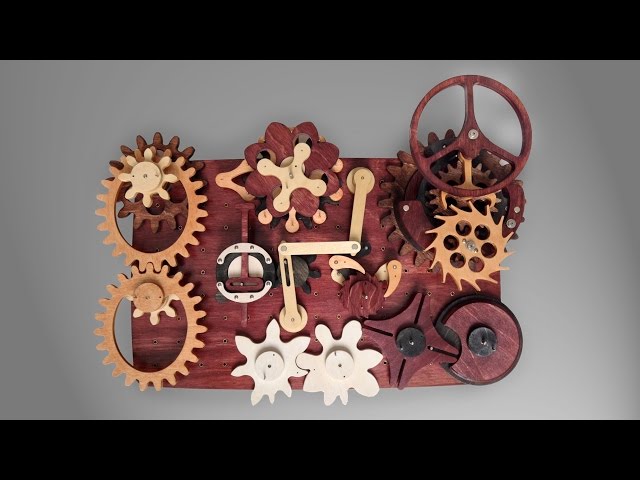The image depicts a playful, machine-like artwork set against a monochromatic gray background. Dominating the center of the composition is a rectangular platform with a reddish hue, filled with an intricate arrangement of various colored gears and mechanical parts. At the top and bottom of the image, there are black horizontal bars that frame the central artwork.

In the lower portion of the artwork, numerous gears of different sizes and colors are visible, creating a cluttered yet intriguing mechanical assembly. There are two white gears at the bottom, positioned next to each other, resembling flowers. To their right are two red gears, one of which features a crescent-shaped cutout that interlocks with the adjacent gear. On the left-hand side, yellow gears are present, adding to the vivid color scheme.

Prominently featured on the upper right corner of the platform is a red circular object resembling a steering wheel. Below this, a cluster of golden, metallic gears is visible, along with a crankshaft that bends at a 90-degree angle. Additionally, the lower left corner showcases an orange gear, paired with a white or cream-colored component.

This detailed mechanical artwork evokes the inner workings of a clock, with its richly colored gears and whimsical design elements blending functionality with visual appeal.